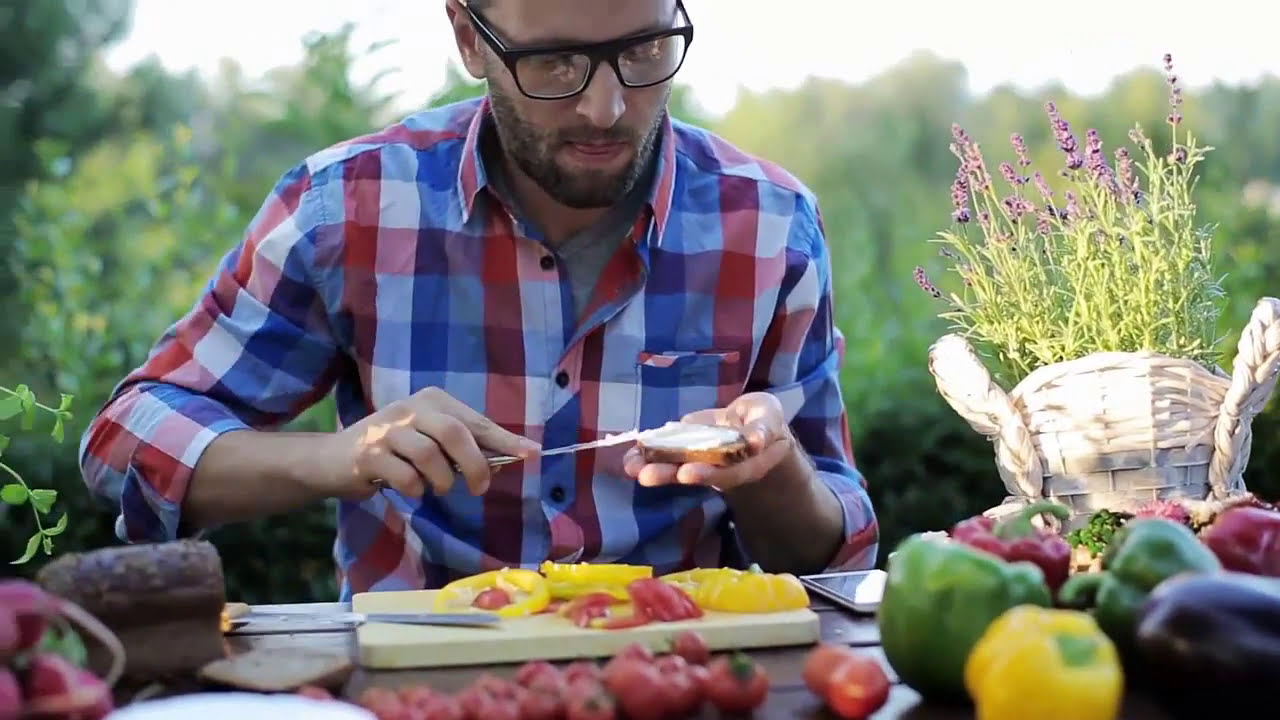In this vivid and detailed outdoor scene, a younger man, sporting a beard and dark-framed glasses, is seated at a picnic table. He is intently focused on spreading what appears to be cream cheese onto a bagel or slice of toast with a knife. The man is dressed in a red, blue, and white plaid shirt, and in the sunlight, his activity is framed by an array of vibrant vegetables and fruits laid out on a wooden cutting board before him. To his right, a lavender plant blooms from a white basket, while a collection of colorful peppers—purple, red, green, and yellow—scatters near petite tomatoes. An eggplant and possibly a loaf of bread, likely the source of his toast, are partially visible as well. The bright, glary sky glows softly in the background, highlighting the lush, blurred foliage that surrounds this serene and bountiful outdoor setting.